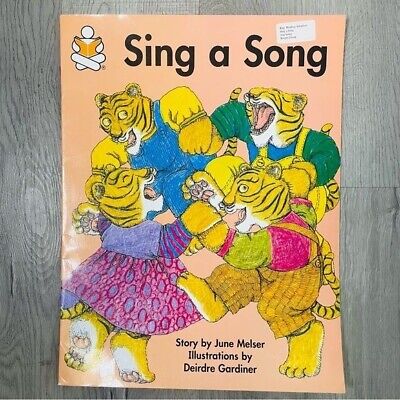This is a square image showcasing the front cover of a children's book placed on a grayish wood surface, possibly a tile, counter, or table. The wood background, featuring a noticeable knot on the left side, contrasts with the book that dominates the center space. The book cover is a light orange or peach color. At the top, in bold black letters, is the title "Sing a Song." Beneath the title, in the upper left corner, there is an outline illustration of a person sitting cross-legged with a book on their lap, reading. The main illustration on the cover features four cartoonish, anthropomorphic tigers, all dressed in various clothes—one in a purple dress, another in brown overalls over a pink shirt, one in overalls over a green shirt, and the last in blue overalls over a yellow shirt. The tigers, depicted as happy and dancing in a circle with linked arms, appear to be singing and enjoying each other's company. At the bottom of the cover, in black text, it reads, "Story by June Melzer, illustrations by Deirdre Gardner."